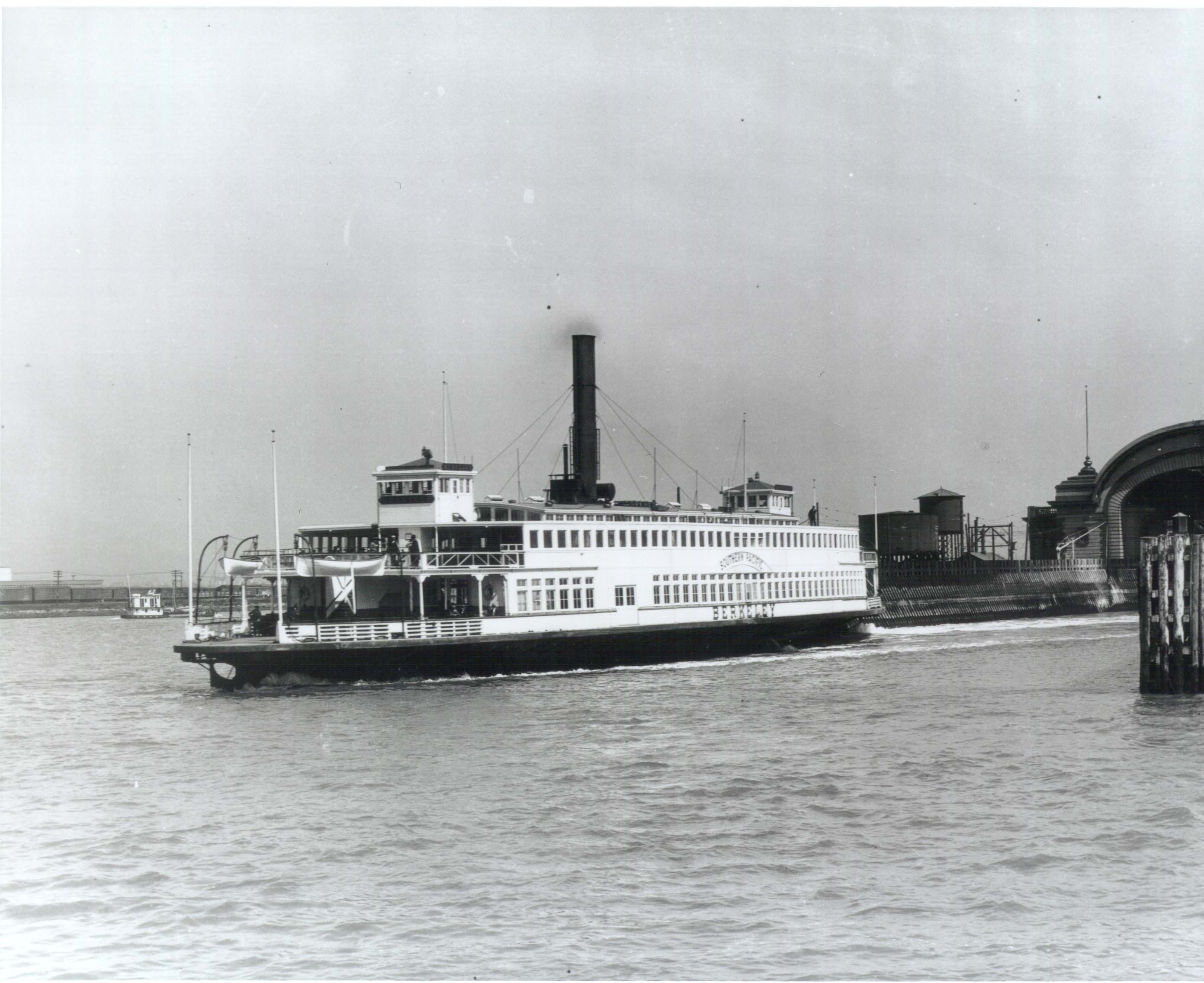This black and white photograph likely from the early 1900s showcases a vintage steam-driven riverboat, resembling a ferry with its elongated design and distinctive features. The boat, named "Berkeley," has the words "Southern Pacific" painted between its rows of windows on the upper and lower decks. The vessel is equipped with a prominent black chimney in the center, indicative of coal-burning steam power, although the paddle wheels typical of such boats are not visible in this image. People are seen on the multiple levels and decks, suggesting it may have been used for both transportation and entertainment. The backdrop includes city structures, such as industrial buildings, a water tower, and a large round structure that could be part of a shipyard, all under a greyish sky. The waterway appears to be a river or large stream, enhancing the historical and utilitarian feel of the scene.